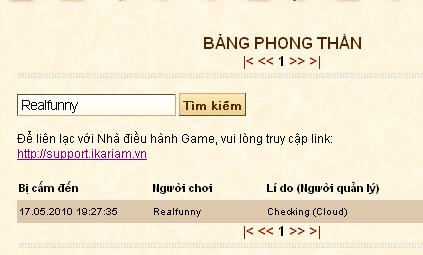This image is a screenshot of a webpage in Vietnamese, characterized by a key search input area and a mix of text and graphical elements. The page title, "Bang Phong Than," is prominently displayed in black in the top right corner. Beneath it is a sequence of lines and arrows with intermittent text, including the number "1". The background is a yellowish-cream color. 

Central to the image is a white input box where "real funny" has been typed, accompanied by a button labeled "Tìm Kiếm" (search). Below this are several sections of black text in Vietnamese, followed by a purple hyperlink to "http://support.icarium.vn." The bottom of the image features a chart with three columns: the first showing numbers, the second repeating "real funny," and the third labeled "checking cloud."

The overall layout suggests a structured form, likely a search interface or ticketing system, with rectangular dimensions. The recurring graphical elements, such as lines and arrows with the number "1" beneath, underscore the orderly design.